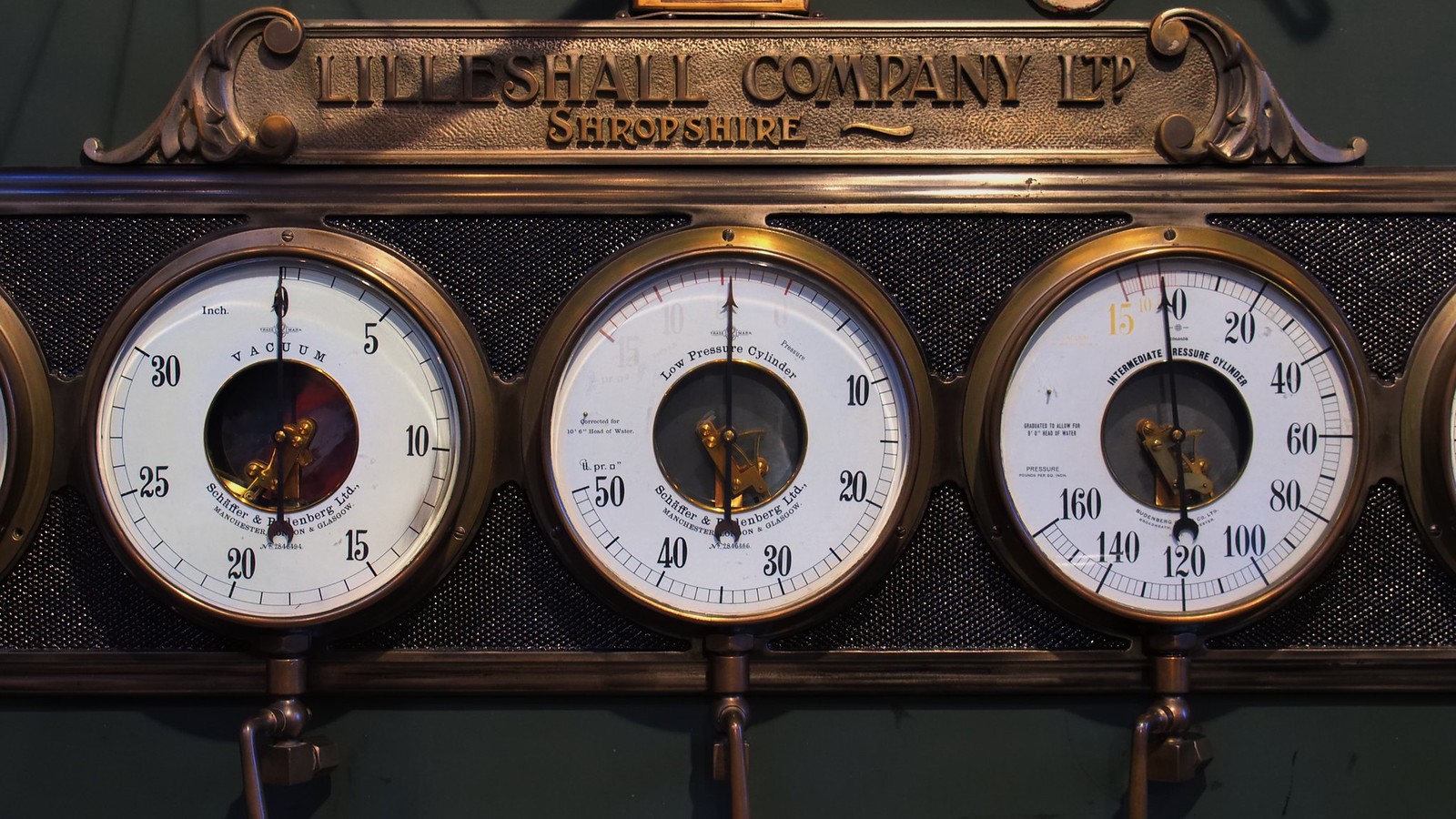The image depicts a metal placard adorned with three 19th-century style pressure gauges. At the top of the placard, encased in a gold-bordered frame, is the label "Lilschall Company LTP Shropshire," presented prominently in capital letters. The three circular gauges below measure different types of pressure. The left gauge, labeled "Vacuum," ranges from 5 to 30. The central gauge, labeled "Low Pressure Cylinder," ranges from 0 to 50. The right gauge, labeled "Intermittent Progressive Cylinder," has a range from 0 to 160. Each gauge features unique numbering, reflecting their specific pressure measurement purposes.